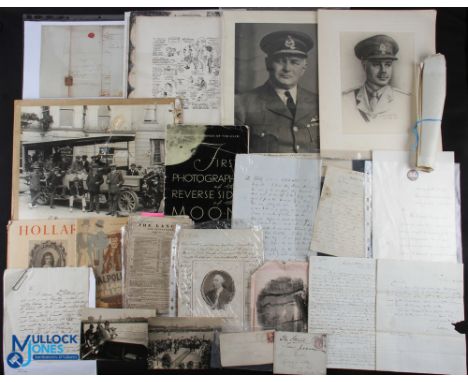The image depicts a meticulously arranged collection of wartime memorabilia, likely from a soldier's service years. Central to the display are various black-and-white photographs, which include portraits of a man in uniform—one from his younger days and another from his older years, both showcasing a hat adorned with a distinctive badge. Surrounding these portraits are additional vintage images, including one of an old-fashioned car surrounded by men in top hats and suits, evoking a sense of a bygone era.

Scattered across the scene are numerous handwritten notes and letters, possibly correspondence exchanged during the war. Some of these notes appear to be heartfelt messages, neatly displayed for viewing. A piece of rolled-up paper tied with a blue ribbon adds a touch of authenticity and nostalgia to the collection. A prominent item in the center is a black book titled "First Photography, Reverse Side of the Moon," hinting at the period's technological and cultural context.

The entire arrangement is set against a dark background, accentuating the monochromatic palette and historical significance of the pieces. This thoughtfully curated assortment captures the poignant memories and personal artifacts of a time long past, offering a glimpse into the life and service of the featured individual.